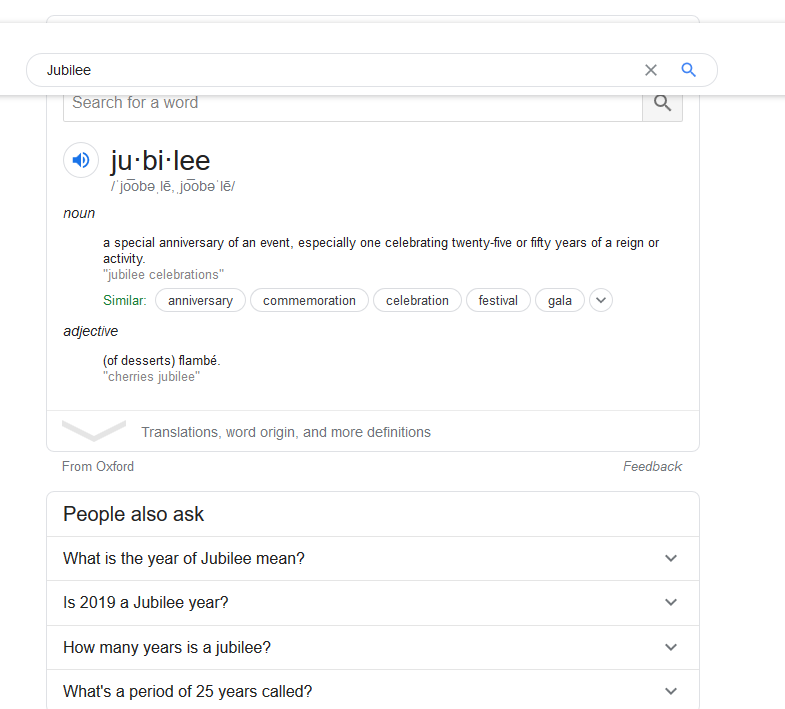Screenshot of Google search results for the term "Jubilee." At the top, the search bar displays "Jubilee" with a capital 'J'. The search bar remains fixed as the user scrolls through the page. The primary definition is provided by Google: "Jubilee" as a noun refers to a special anniversary, particularly one celebrating 25 or 50 years of an event, reign, or activity. It includes an example usage: "Jubilee celebrations" and lists similar terms such as anniversary, commemoration, celebration, festival, and gala. 

The secondary definition pertains to the adjective form, specifically in the context of flambé desserts, exemplified by "cherries Jubilee." Below the definitions, there's a faint downward arrow indicating links for translations, word origin, and more definitions, with credit attributed to Oxford. On the left, a blue audio icon is available to hear the pronunciation of "Jubilee." To the right, a feedback option is presented. Further down, the "People also ask" section provides four related questions: "What does the year of Jubilee mean?," "Is 2019 a Jubilee year?," "How many years is a Jubilee?," and "What's a period of 25 years called?"